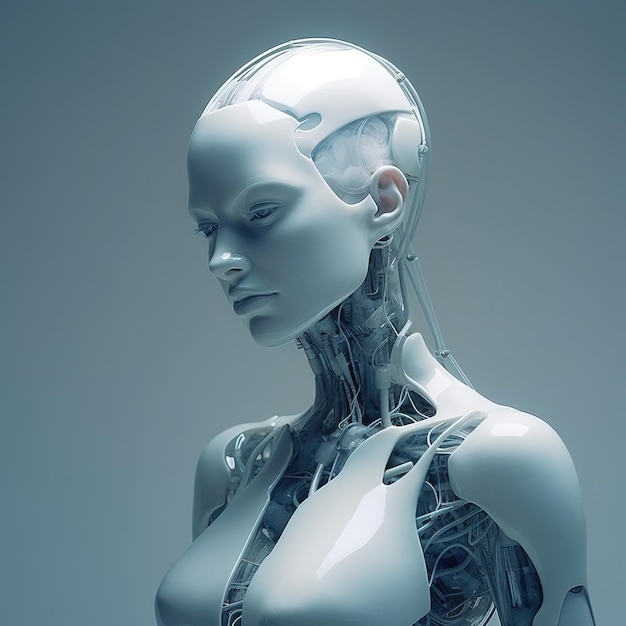The image depicts a detailed, white, female-like robotic figurine set against a dark gray background. The android's body, from its breasts up, is primarily composed of opaque white plastic plates with a sheen, covering her face, chest, and shoulders. The plates are meticulously designed to mimic a female form, including distinct facial features and a female-like structure. The figurine's expression is neutral, with open eyes and no eyebrows, while her head showcases ears on both sides and a translucent section revealing a complex network of wires and compartments. Through the transparent sections of her body, one can see an intricate internal structure of interconnected wires and perhaps some simulated arteries and veins, adding a layer of depth to the mechanical intricacy. The back of her head is also exposed, further showcasing the blend of external structure and internal mechanics. Overall, the image illustrates a highly sophisticated and sterile representation of a female android, focused on emphasizing both the external human-like features and the revealed internal components.